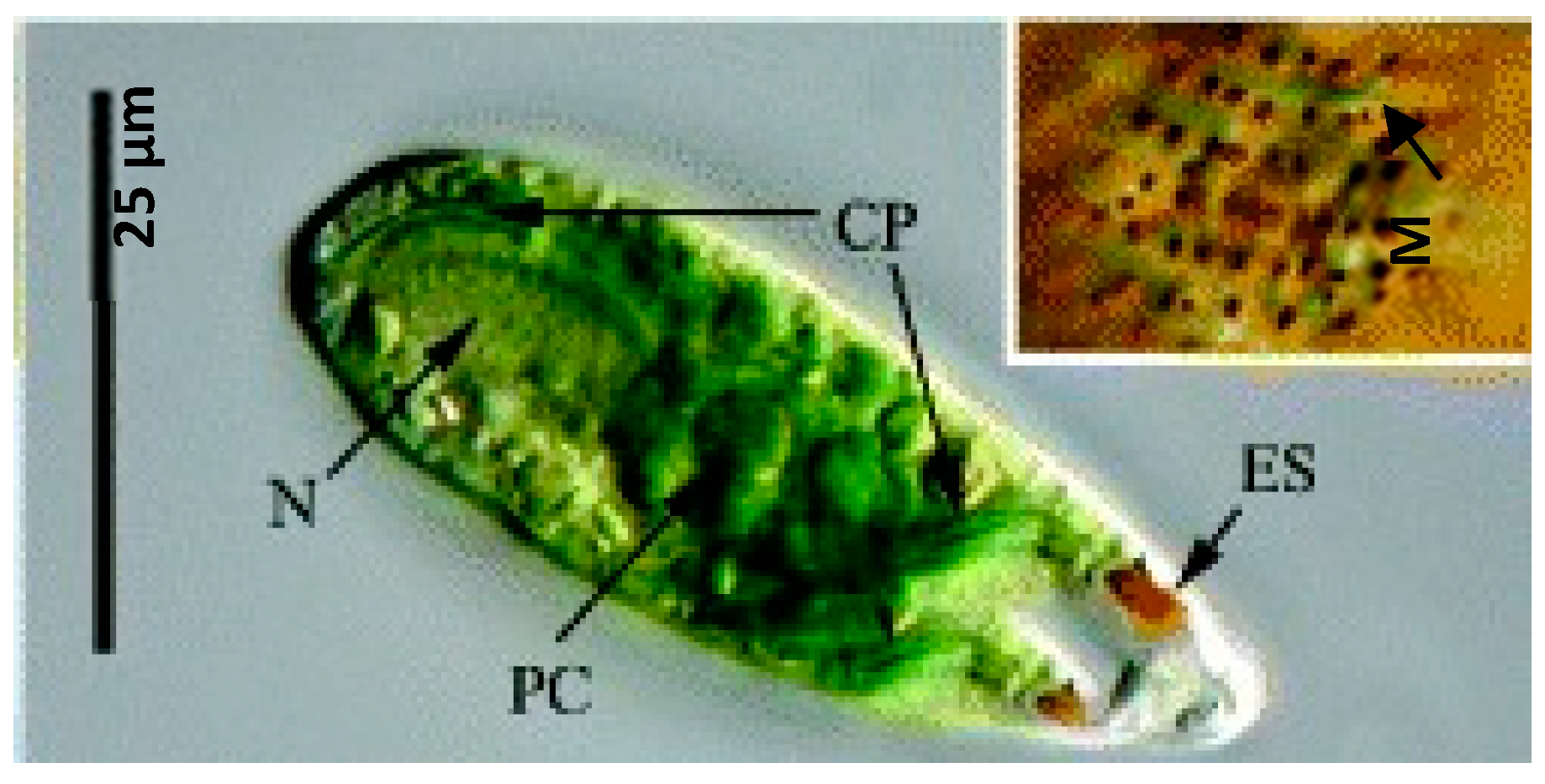This is an image, possibly a computer-generated representation or a photograph, that appears to depict a microscopic organism, akin to an amoeba or perhaps a plant cell. The organism is predominantly green, with occasional highlights of yellow and orange, set against a bluish-gray background. Its overall shape is oval. The image quality is somewhat fuzzy and pixelated, suggesting it is a high-magnification view.

The diagram includes various labeled arrows pointing to key parts of the organism, with annotations such as N, PC, CP, and ES. Notably, one label suggests the presence of eye-like structures. Additionally, there is a vertical scale bar on the left side of the image marked "25" with some unclear symbols, indicating the measurement scale. In the top right corner, there is an inset showing a detailed area of the organism's structure, featuring black dots against a brown and tan background with green elements, labeled as "M." The inset provides a zoomed-in view of a specific aspect of the organism but does not include further explanation.